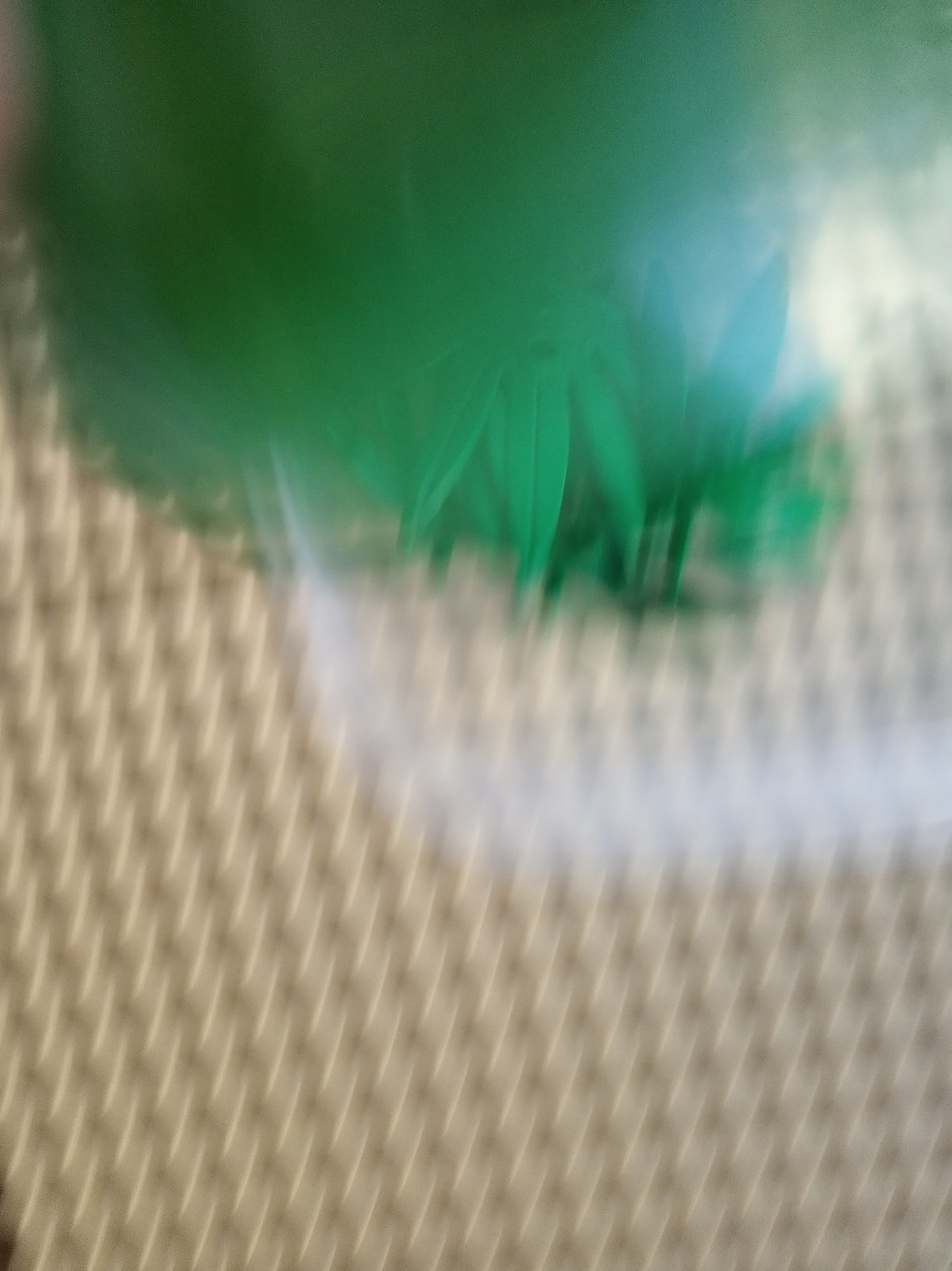This photograph, though blurred, captures a plant with elongated, pointy leaves that appear to radiate from a central stem. Each stem seems to cluster around eight distinct leaves, giving it a starburst-like formation. The plant is housed in what looks like a clear plastic Tupperware container, allowing a glimpse of its resting place. Natural light from the right-hand side illuminates the plant and container, casting soft shadows and highlighting the texture of the leaves. The scene is set atop a gingham-patterned tablecloth featuring a palette of light brown, tan, and dark brown hues. Notably, the upper left corner reveals some shadowing, indicating additional light sources or objects outside the frame.